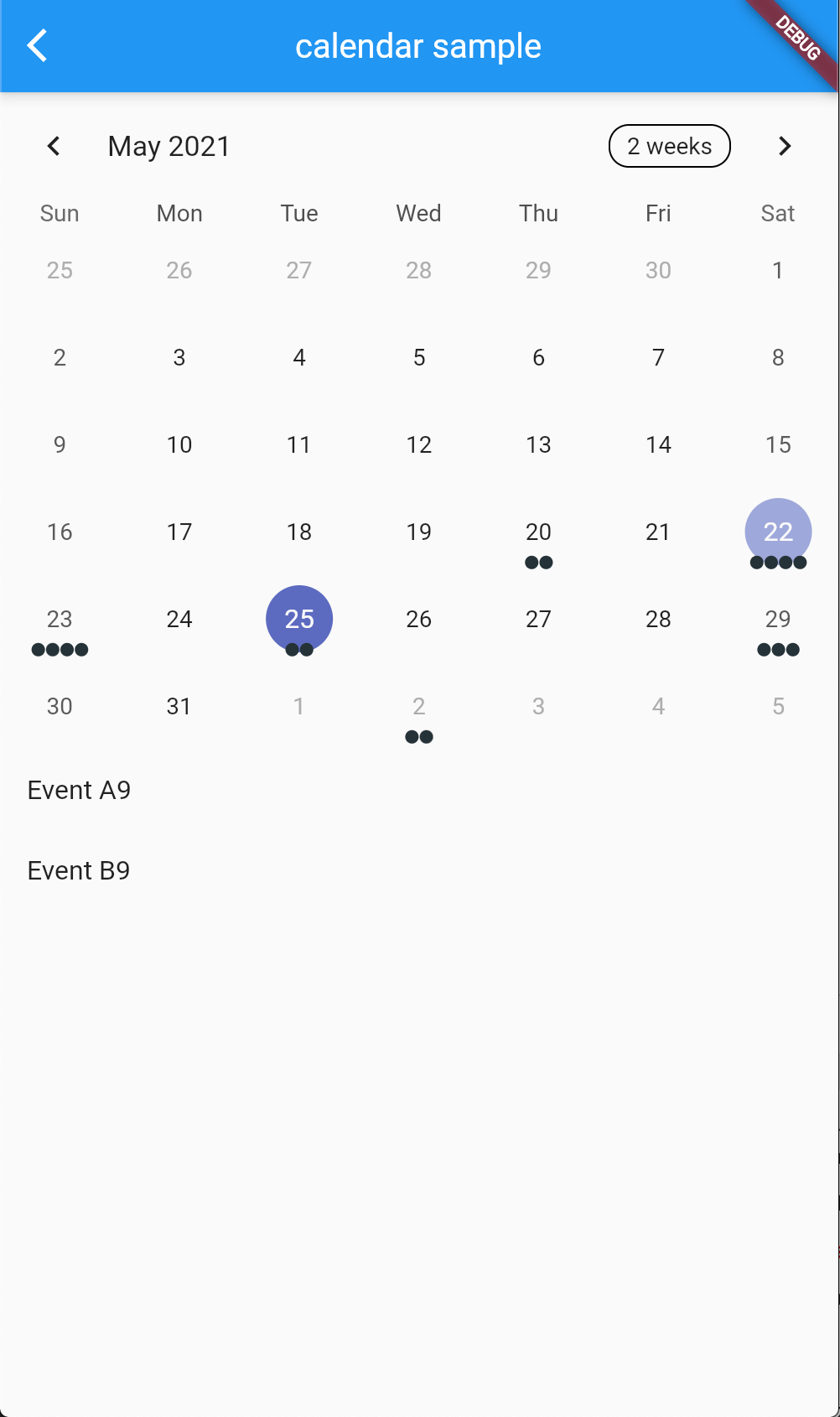This image is a plain, basic screenshot of a calendar interface. At the top of the screenshot, there's a navigation bar that includes a back arrow on the left and, in white lowercase text resembling Times New Roman, the words "calendar sample." On the right side of this colored bar, there's a maroon banner with the word "DEBUG" in white capital letters.

Below the navigation bar is a standard monthly calendar view for May 2021. To the left of the calendar view, there's another back arrow to navigate back to the year view. To the right, a circled label reads "two weeks," likely a shortcut to switch to a two-week view.

The calendar itself features a black font on a white background. Specific dates are highlighted: May 22nd has a light blue ring with four black dots underneath it, while May 25th has a darker blue ring with two black dots. Other dates with black dots under them include May 20th, May 23rd, May 29th, and June 2nd, each indicating different events or reminders.

Underneath the calendar, two event entries are listed: "event A9" and "event B9," both written in the same unbolded Times New Roman-like font.